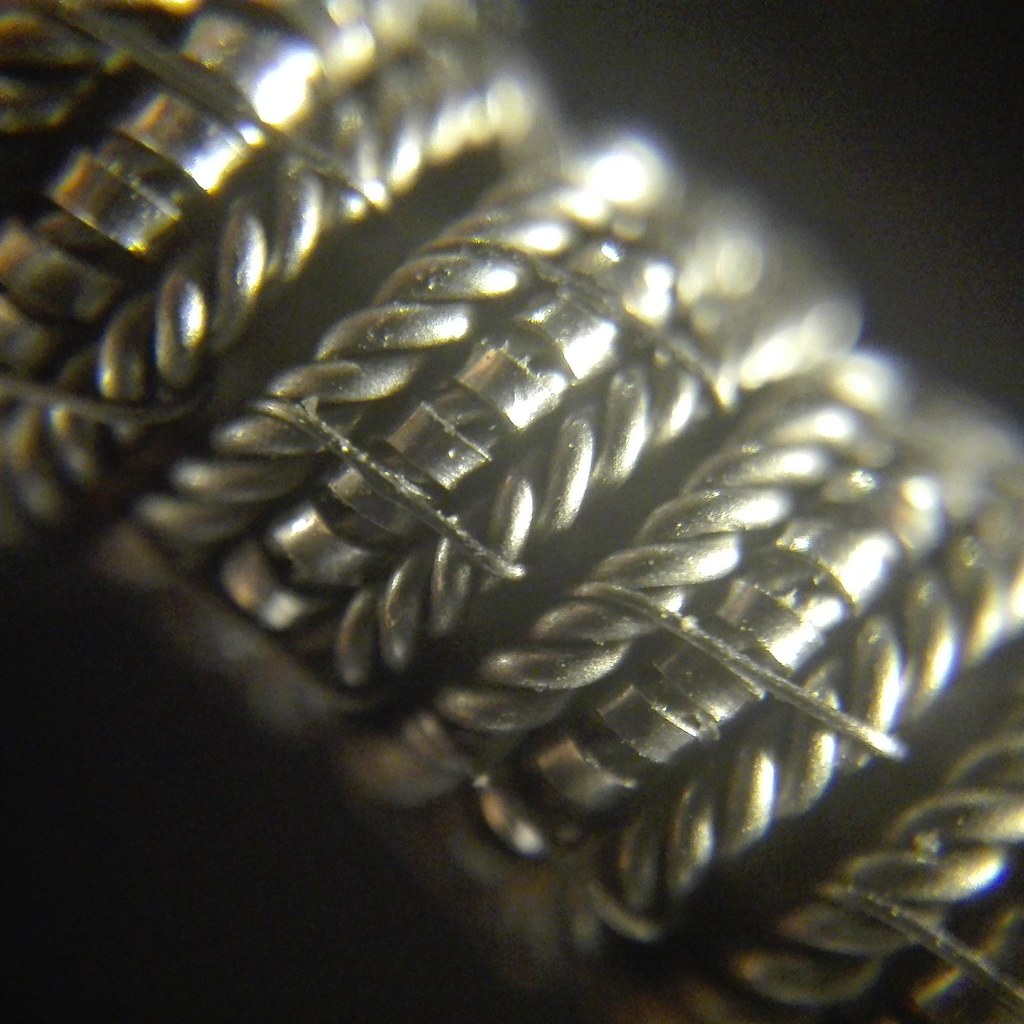The photograph is an extreme close-up, almost microscopic, of an intricately detailed object that appears to be a piece of jewelry. The image predominantly features multiple bands of gold, coiled in a helical pattern, which run diagonally from the back right to the bottom left. Each band is composed of three intertwined strands of gold; the middle strand is interspersed with small, horizontal buckles or bands, and contains visible threads or cores. Though the specific object that these bands encircle is obscured by shadow and remains unidentified, the bands create a circular formation. The top sections of the bands, towards the top right corner, are blurred, focusing on the foreground. Highlight reflections indicate a light source from the lower right. Despite some descriptions suggesting a silver hue, the prevailing details confirm the material as gold.